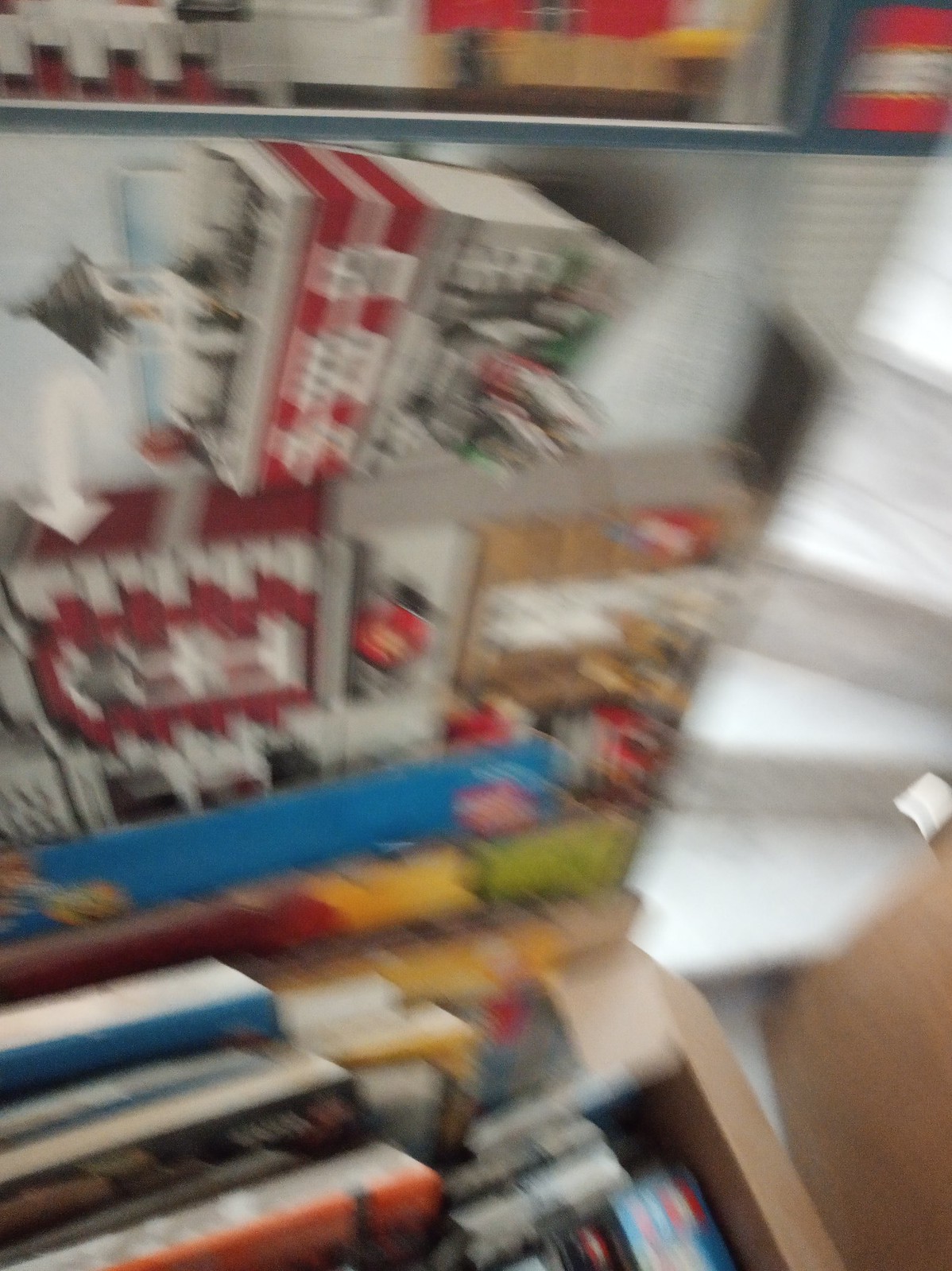This indoor image captures a somewhat blurry retail store display, making detailed observation challenging. 

To the left, there's a display rack filled with various products, possibly candy, gum, or cigarettes. The items exhibit a mixture of colors including patches of green, yellow, and red, with red and white packages prominently placed on the top shelf. 

On the right side of the photo, white-painted stairs ascend, adding a structural element to the scene. 

Additionally, a top shelf spans the upper section of the image, holding more indeterminate boxes or packages.

Overall, the photograph presents a slightly out-of-focus view of a store's product area and architectural features.